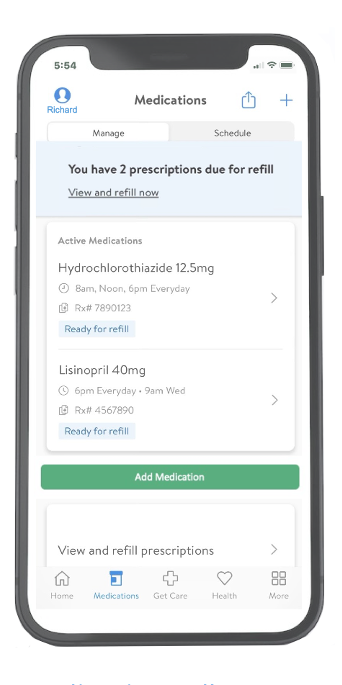The image depicts a mock-up style screenshot of a phone's front screen, showcasing a pharmacy or prescription refill application. The phone, with a black frame, is set against a white background. At the top of the screen, the standard phone UI elements are visible, including the time, signal strength, Wi-Fi connection, and battery icon, all in black. 

The main content area features a white background. Near the top, the word "Medications" is prominently displayed in black text, followed by a circle icon on the left side which likely signifies the logged-in user’s profile. The user is identified as "Richard" in blue text. On the right side of "Medications", there are two icons: an exit symbol and a plus sign for adding new items.

Below this section, two tabs are visible: "Manage" on the left with a white background, and "Schedule" on the right with a light gray background, indicating different sections of the app.

In the next section, a bluish-gray background rectangle states, "You have two prescriptions due for refill," followed by a clickable prompt "View and refill now."

Following this, the active medications are listed in a structured format:
1. **Hydrochlorothiazide 12.5 mg**:
   - Displayed within a white background box with a slight shadow.
   - Includes a clock symbol indicating dosage times: 8 a.m., Noon, and 6 p.m. daily.
   - Rx number: 7890123.
   - A blue rectangle labeled "Ready for refill" to the right, indicating action availability.
   - A grey line separates this medication from the next.

2. **Lisinopril 40 mg**:
   - Presented similarly with dosage times, Rx number, and a "Ready for refill" button.
   - Set within a slightly curved box with a shadow effect.

Below the medication list, a large green button spans the width of the screen with rounded corners, labeled "Add Medication" in white text.

At the bottom, a partially cut-off white box with curved edges and a shadow provides additional options with a link saying "View and refill prescriptions" followed by a greater-than symbol.

The app's navigation bar is positioned at the bottom of the screen:
- **Home**: with a home icon.
- **Medications**: with a medicine bottle icon.
- **Get Care**: with a medical cross icon.
- **Health**: with a heart icon.
- **More**: with a grid of four squares icon.

The detailed layout and labels suggest a user-friendly interface designed to manage and refill prescriptions effectively.